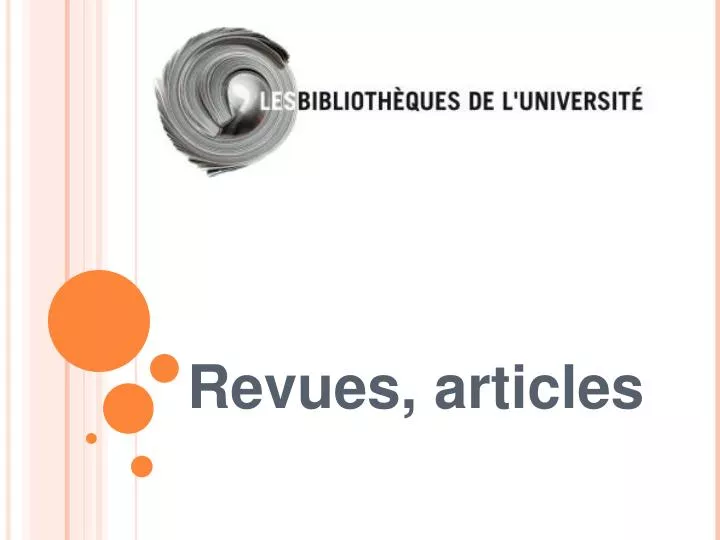The image features a predominantly white background. On the right edge of the image, a single thin orange line descends from top to bottom. On the left side, there's a wider pale orange stripe accompanied by four additional vertical lines of varying orange hues. Positioned centrally at the top of the image, a textured black swirl curves counterclockwise, starting from just right of the center. To the right of this swirl, the text "LES BIBLIOTHÈQUES DE L'UNIVERSITÉ" is displayed, with "LES" in white block letters and the rest in black block print. The second 'E' in "BIBLIOTHÈQUES" features an accent mark curving from the top right to the bottom left, while the final 'E' in "UNIVERSITÉ" has an accent mark curving from the top left to the bottom right.

Beneath this text, more towards the lower section, two gray words are displayed: "REVUES, articles," with the 'R' in "REVUES" capitalized, and the rest in lowercase. To the left of these words, there are five orange circles forming an irregular pattern resembling an imbalanced five-pointed star. The largest circle is situated near the top left, with progressively smaller circles arranged diagonally downwards and slightly to the right, and one additional smaller circle placed to the left of the second-largest one. These circles and lines contrast against the white background, creating a visually engaging composition.